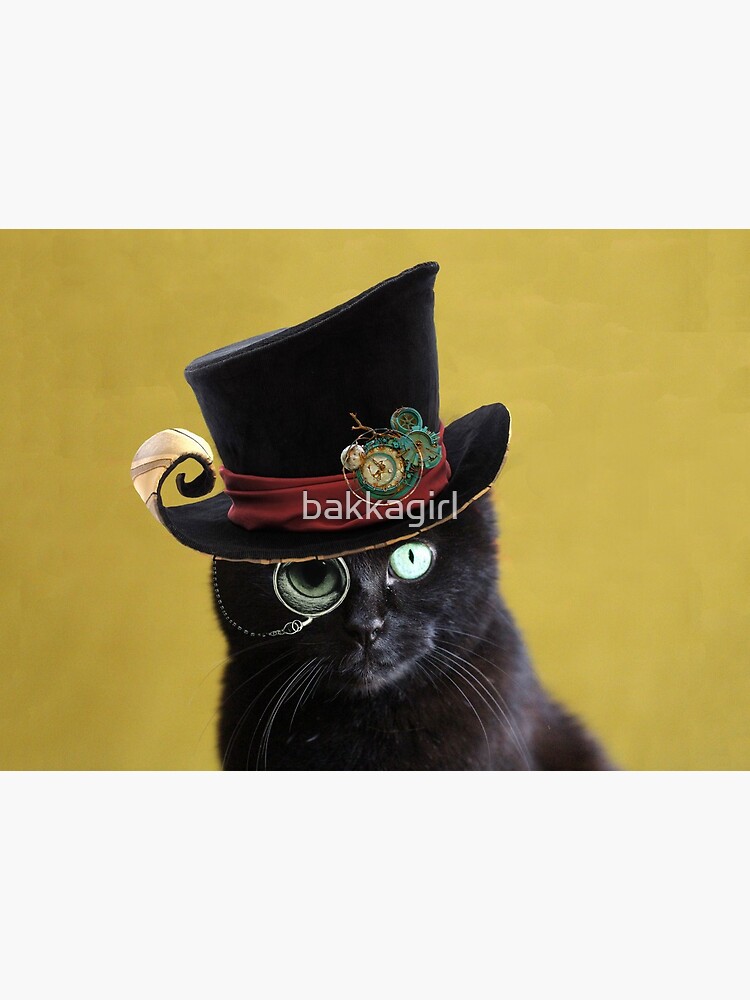A sophisticated black cat dons a steampunk-inspired top hat and monocle. The top hat, adorned with a wine-colored band and a white feather, boasts intricate clock gears at its curled brim, leading up to a pointed peak. The cat's sleek black fur contrasts beautifully with its gleaming green eyes, one of which is magnified by the monocle. Its long whiskers hang elegantly, framing its calm and composed expression. The background, a muted blend of greenish-yellow, further accentuates the cat's refined appearance.